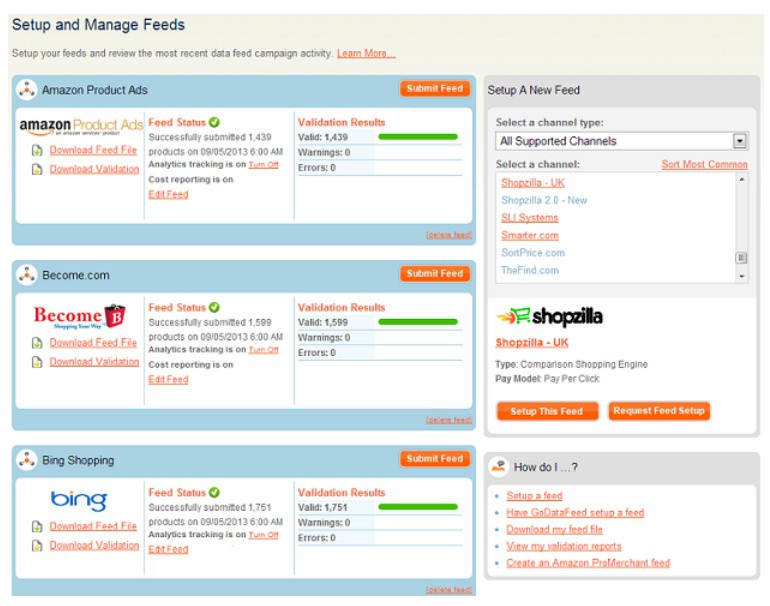**Detailed Caption for the Image:**

In the upper left corner of the image, the text "Set Up and Manage Feeds" is displayed prominently. Directly below this heading, a subheading reads, "Set Up Your Feeds and Review the Most Recent Data Feed Campaign Activity." An underlined "Learn More" in red is situated below the subheading. This entire section is set against a light tan-colored background.

Beneath this introductory information, the image transitions into three distinct rectangles, each having a light gray-green color. 

- The first rectangle at the top contains detailed status information about an Amazon Product Ad feed. It includes multiple elements:
  - **Headings**: "Amazon Product Ad" and "Amazon Product Ads."
  - **Links and Actions**: "Download Feed File" and "Download Validation."
  - **Status Indicator**: A green check mark inside a circle with the text "Successfully Submitted 1,439 Products on 9-5-2013 at 6 a.m."
  - Additional Options: "Analysis Tracking is on" with "Turn Off" underlined in red, "Cost Reporting on," and "Edit Feed" in red.
  - **Validation Results**: A green bar indicating "Validated 1,439" with another section for warnings and errors showing "Warning Zero" and "Arrow Zero."
  - **Submission Action**: An orange button labeled "Submit Feed" above these fields.

- The second rectangle follows a similar format but pertains to the BECOME feed:
  - **Headings**: "BECOME" (with the acronym spelled out as B-E-C-O-M-E).
  - **Status Indicator**: "Successfully Submitted 15,099 Products on 9-5-2013 at 6 a.m."
  - Additional Options: "Analysis Tracking is on," "Cost Reporting is on."
  - **Validation Results**: A green bar indicating "Validated 1,599."

- The third and final rectangle is dedicated to Bing. It abbreviates key information while retaining the same formatting style as the previous two sections.

Each section's uniform design provides a comprehensive overview of the feed management status across different platforms.